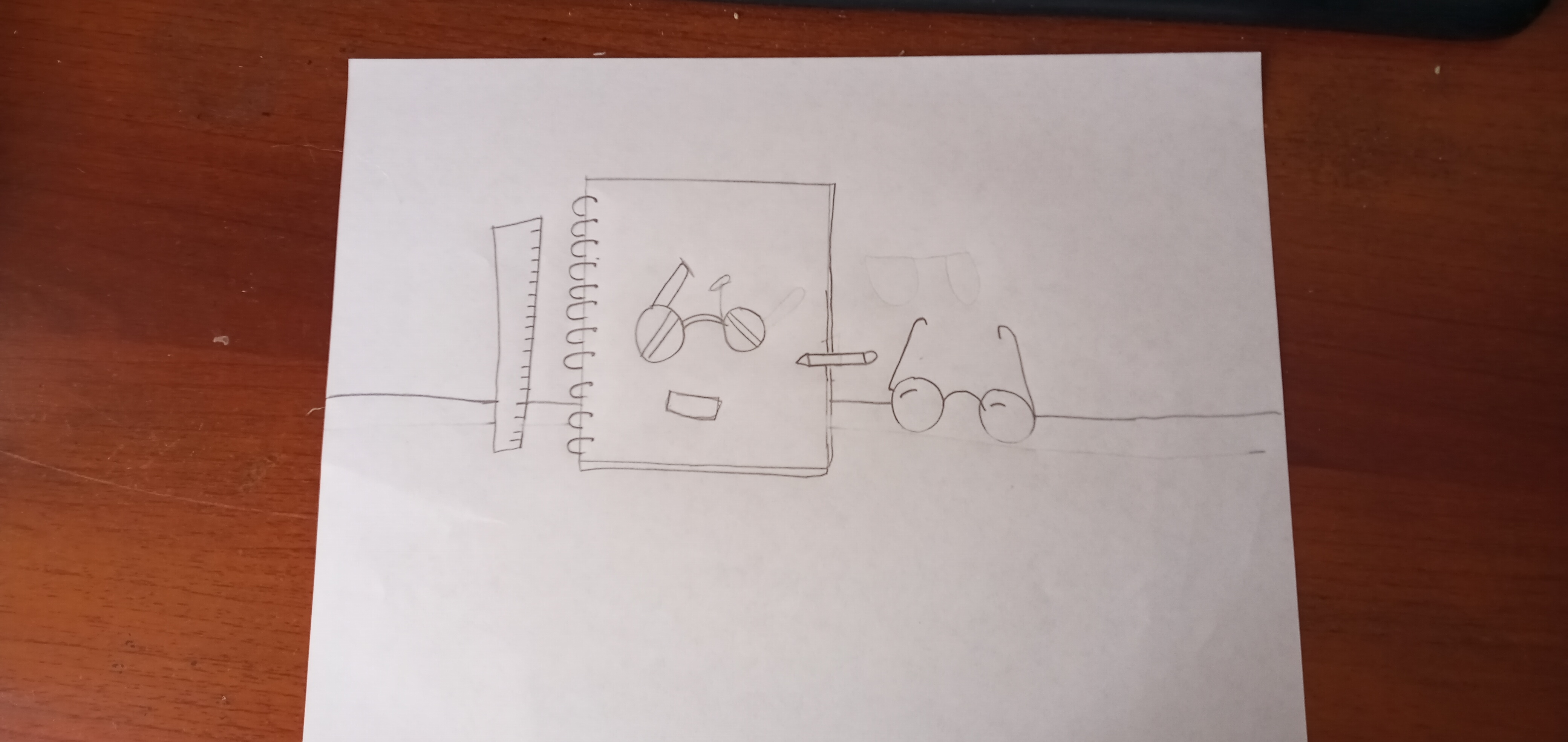The photograph captures a standard 8.5 by 11-inch white sheet of copy paper, meticulously placed at the center of a solid oak desk with a reddish-brown tint. Drawn in pencil, creating a monochromatic composition, a single horizontal line runs through the center of the paper. Along this line, various school items are neatly sketched. To the far left, a vertical ruler stands prominently. Adjacent to the ruler, a spiral notebook is illustrated with whimsical detail, featuring a face complete with glasses and a smiling mouth. Following the notebook, a pair of round glasses is carefully rendered, adding charm to the collection of school-themed drawings. The oak desk's grain and rich hue contrast subtly with the simplicity of the pencil artwork, creating an engaging visual narrative.